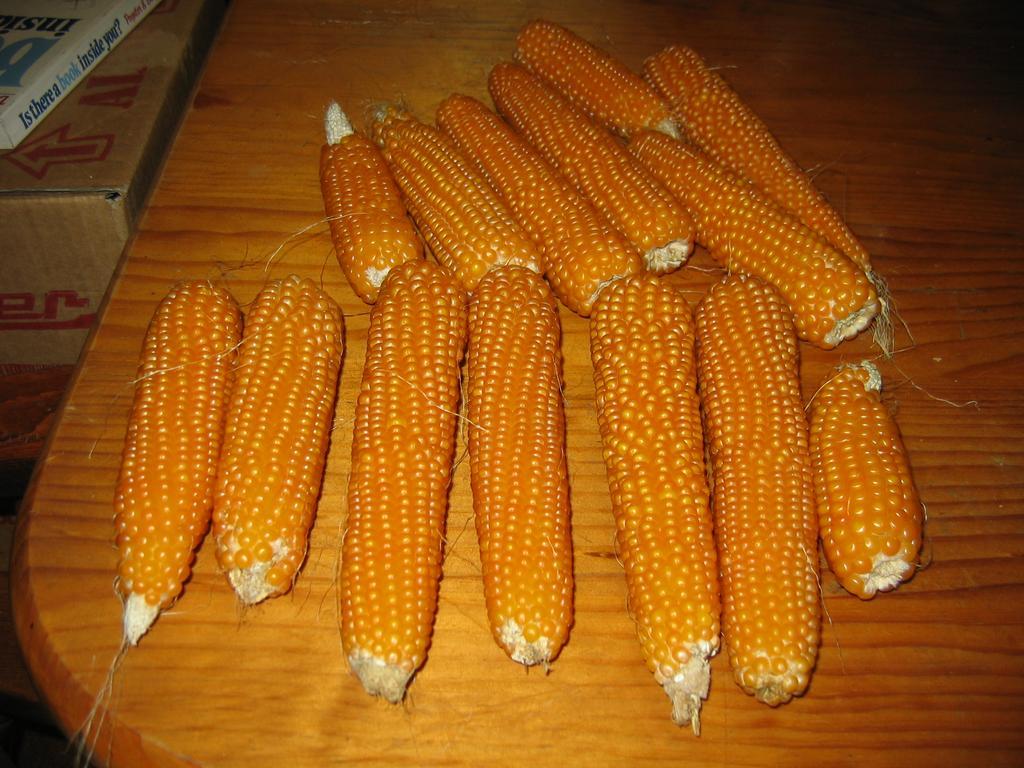The photograph displays 14 dried ears of yellow corn neatly arranged on a wooden table with rounded corners. The corn, devoid of husks and outer layers, exhibits a golden yellow color with shiny kernels, indicative of its dried state, often referred to as Indian corn. The ears vary in size, with some being short and nubby while others are longer and skinnier, occasionally retaining pieces of the stalk at the ends. In the upper left corner of the image, a cardboard box with red print is visible, topped by a paperback book titled "Is There a Book Inside You?" The arrangement of the corn suggests two rows with the front row comprising seven distinguishable ears. The scene captures the rustic charm of autumnal harvests, with the detailed textures of the corn and the wooden table adding to the visual appeal.